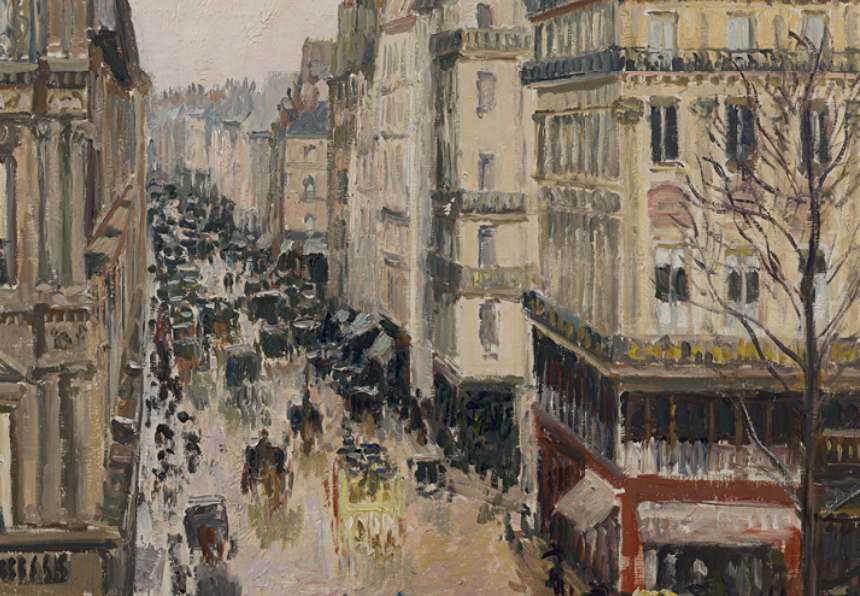This rectangular, horizontally oriented painting depicts a vibrant city street scene viewed from an elevated perspective, possibly the third or fourth level of a building, or even a bird's-eye view. Rendered in an impressionistic style, the painting utilizes tones of tan, brown, yellow, and orange for the multi-story masonry or concrete buildings that line both sides of the street. The bustling thoroughfare down the center of the scene is teeming with black horse-drawn carriages or buggies, creating a high traffic, boisterous atmosphere. A tree in the foreground to the right adds a touch of greenery to this busy, lively scene.